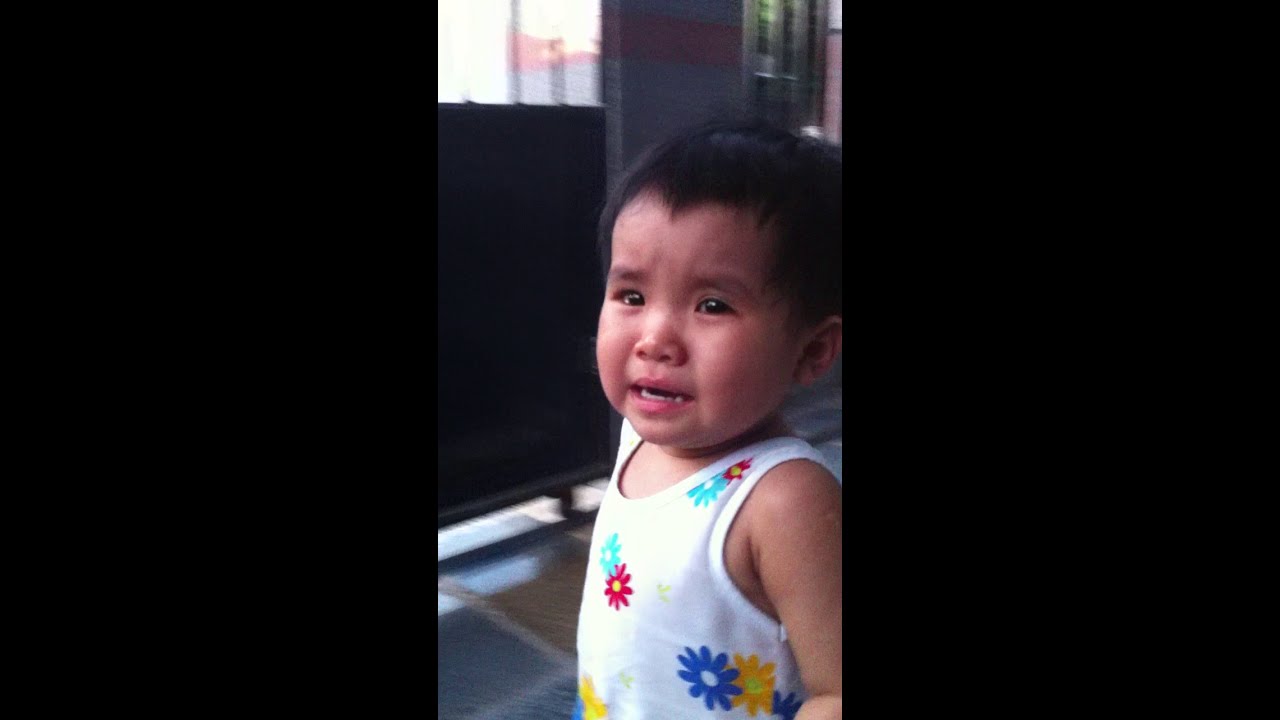In this image, we see a very young boy, approximately between one to three years old, who appears either to have just started crying or to have just finished. His short hair and fully grown white teeth are visible. He is wearing a sleeveless, white tank top adorned with various colorful flowers. The flowers display a range of colors including teal, red, blue, yellow, royal blue, and bright gold. Notably, there is a red and teal flower on his left shoulder, a blue and yellow flower under his armpit, and a yellow flower on his belly, paired with part of a blue or teal flower. The setting seems to be indoors, likely inside a living room, given the light blue and light yellow tiled floor, although the image is somewhat dark. The boy stands slightly to the right of the image's center, looking towards the camera with an upset expression. The left and right sides of the image feature black rectangular borders, contributing to a frame-like appearance. The background is blurry, obscuring specific details about other objects present. The varying colors in the image include black, gray, brown, light blue, red, white, green, tan, and pink.